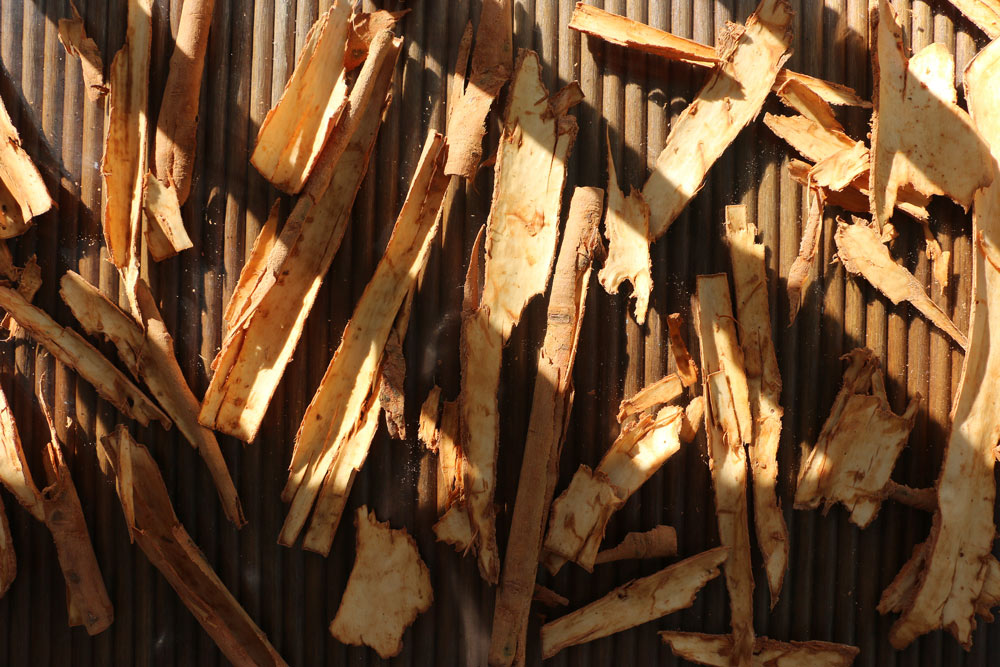In this horizontal rectangular outdoor image, the focal point is a weathered wooden or bamboo stick fence, composed of long, thin poles that span the height and width of the frame. The brown-colored fence serves as the backdrop, with sunlight illuminating parts of it, particularly in the upper right corner, while shadows traverse diagonally across the scene. Scattered across the surface of the fence are numerous wood shavings and pieces of bark, revealing the inner, smooth layers and the outer, rough texture of the bark. These wood fragments, ranging from rounded to straight, are strewn all over, creating a scattered, almost chaotic, pattern. The lower left corner of the image is noticeably darker, likely due to the shadows cast by the fence, adding contrast to the otherwise sunlit composition.